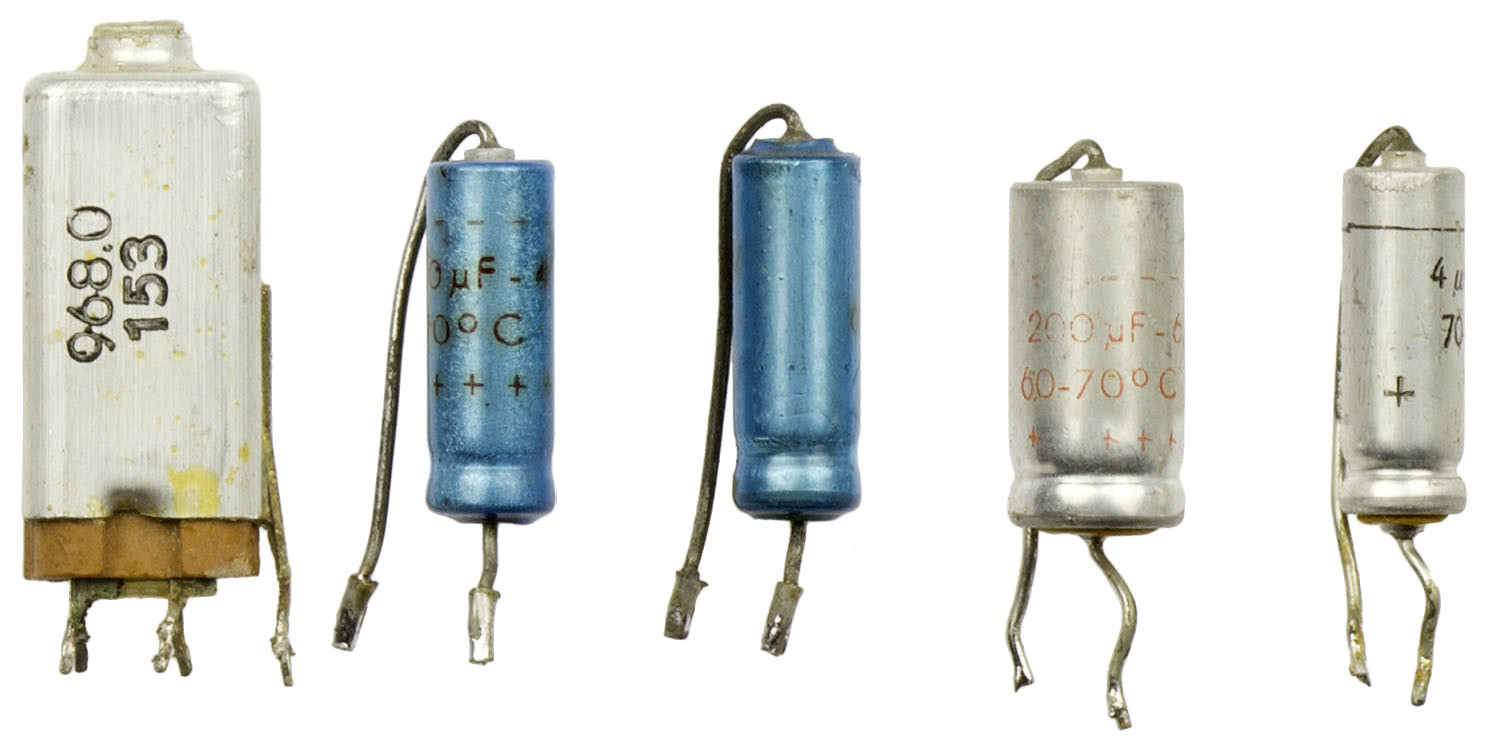The image displays five vintage tube amplifiers, often used in old radios. The first amplifier on the far left is notably the largest and has a silver square top with the numbers "968.0153" printed vertically. It transitions to a brass base and features two prongs at the bottom and one on the side. Next to it are two smaller blue amplifiers that look almost identical; the first of these has the label "OUFOOC" along with a black wire emanating from the top and a silver wire from the bottom, indicating the negative and positive sides. The second blue amplifier, similar in design, lacks any writing but also has wires coming out from both the top and bottom. The fourth amplifier is a wider silver cylinder with orange writing that reads "200UF - 660 - 70 C" and indicates the negative and positive sides. It also has wires extending from both the top and bottom. The final amplifier is a smaller silver cylinder, featuring partially visible black writing, possibly showing "4" and "70," with analogous wiring conventions. These tube amps, with their wires and labeled prongs, hint at components used in historical electronic equipment.